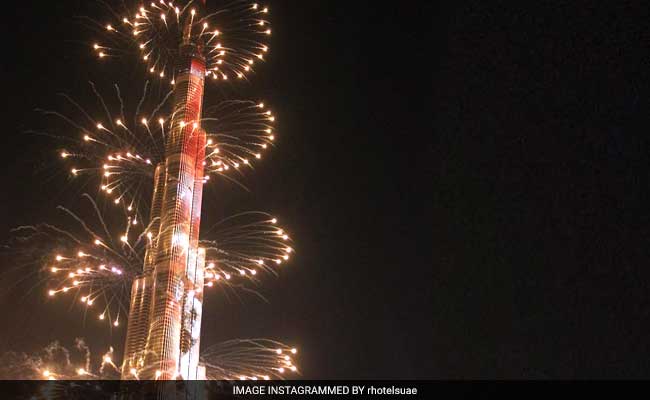The image features the iconic Burj Khalifa in Dubai, the tallest building in the world, captured on a black night sky backdrop devoid of stars, likely due to light pollution. The Burj Khalifa stands prominently on the left side of the frame, its glass exterior reflecting hues of red and white. A spectacular display of fireworks wraps around the building in a helical pattern, starting from the base and spiraling upward, their bright yellow bursts illuminating the otherwise dark scene. The entire building is breathtakingly lit up by this vivid firework display. At the bottom center of the image, bordered by a darker black, is a caption in white text that reads "Image Instagrammed by Rotel Suet."